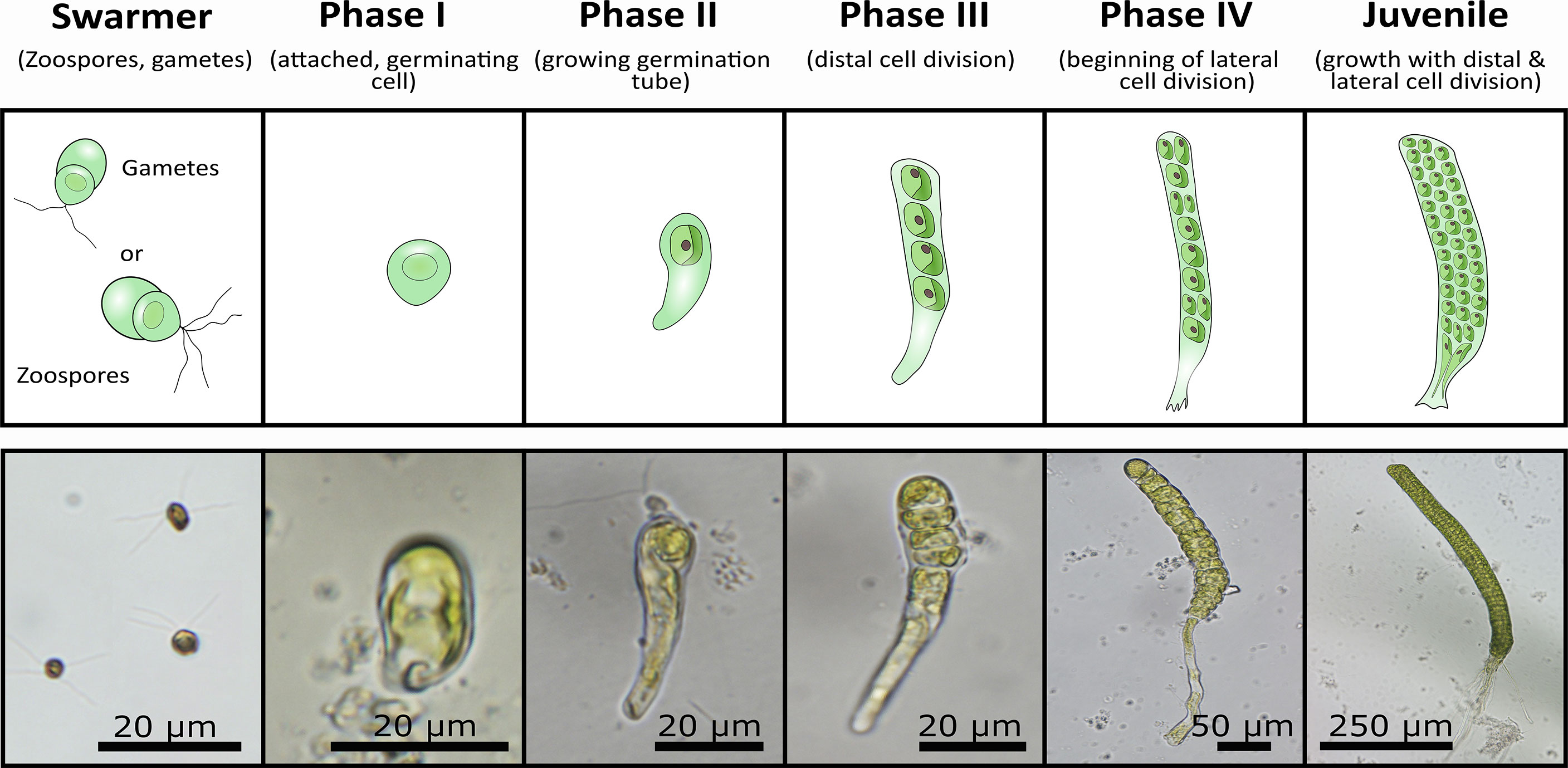The image is a landscape-oriented chart illustrating the phases of cell division through graphical and real-life microscopy representations. It is divided into six columns, each representing a different phase labeled at the top: Swarmer, Phase I, Phase II, Phase III, Phase IV, and Juvenile, with respective Roman numerals. Each column features two rows; the top row displays cartoon depictions on white backgrounds, while the bottom row presents electron microscope images with greyish-brown backgrounds and scale indicators.

From left to right:

- **Swarmer:** Depicts gametes or zoospores, shown as green circles with tendrils.
- **Phase I:** Attached germinating cell, illustrated by a single green circle.
- **Phase II:** Growing germination tube, showing a bean-like shape with a green circle and red dot inside.
- **Phase III:** Distal cell division, depicted as a stalk with multiple green circles and red dots.
- **Phase IV:** Beginning of lateral cell division, with numerous dots and circles increasing in number.
- **Juvenile:** Growth featuring both distal and lateral cell division, culminating in about 30-40 cell representations.

The cartoon cells feature additional textual descriptions like "gametes" or "zoospores," while the microscopy images provide scale measurements ranging from 20 μm to 250 μm. The 250 μm scale is uniquely positioned at the bottom left, whereas the others are in the bottom right of their respective images. This chart provides a clear, detailed visual comparison between cartoon illustrations and real electron microscope images of the cell division process from swarmer cells to juvenile stages.